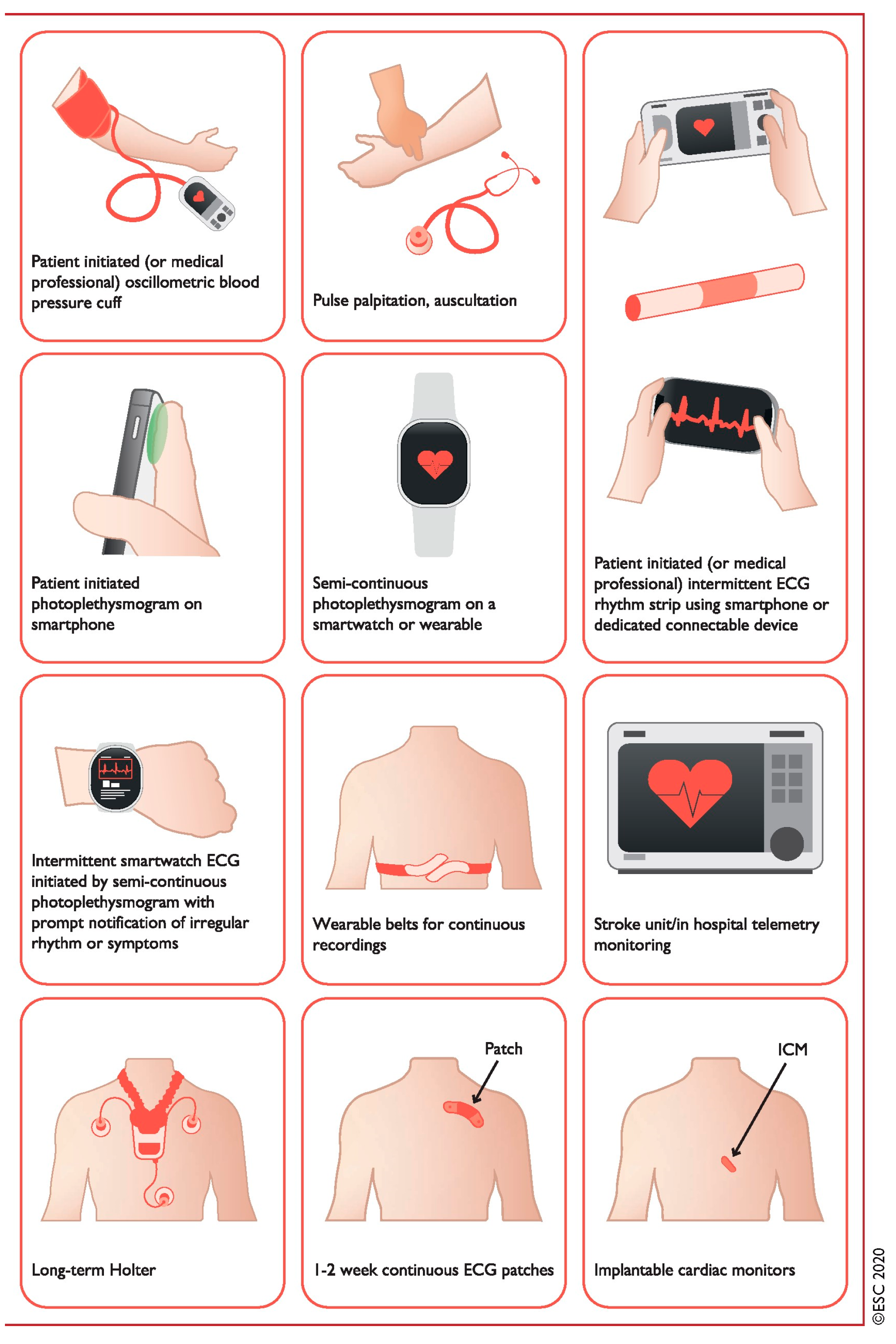This detailed descriptive caption synthesizes the key elements from all three users, focusing on the repetitive and shared information while elaborating on the visual content and context:

---

The image features a detailed medical infographic set against a solid white background, consisting of twelve individual boxes, each illustrating various medical devices and procedures related to heart monitoring and critical care. The top left box depicts a red cuff on the right arm for measuring blood pressure, labeled "Patient-initiated or medical professional osculometric blood pressure cuff." Moving to the right, the next image shows a person interacting with a device, labeled "Patient-initiated or medical professional intermittent ECG rhythm strip using smartphone or dedicated connectable device." Continuing to the right, we see a photo of a thumb against a smartphone with a green highlighted area, indicating a "Patient-initiated photoplethysmographic mammogram on smartphone."

Beneath this, there's an image of a white smartwatch with a black screen displaying a red heart, described as a "Semi-conscious photoplethysmographic mammogram on smartwatch or wearable." The left side shows another image of an arm with a watch, illustrating an "Intermittent smartwatch ECG initiated by semi-conscious individual, with prompt notification of irregular rhythm or symptoms." Further down, a back view features a belt for continuous monitoring, and an adjacent image represents hospital telemetry monitoring in a stroke unit, symbolized by a heart inside a microwave-like graphic.

On the bottom left, there's a depiction of a torso with a red object on the chest and three stickers, labeled "Long-term Holter monitor." The next image shows a red bandage-like patch on the shoulder blade, indicating "One-to-two week continuous ECG patches." Finally, the bottom right illustration highlights an "Implantable Cardiac Monitor," marked by a small red dot on the back of an individual. Each of these hand-drawn images serves as an instructional guide, primarily showcasing self-monitoring medical devices and techniques for managing heart conditions such as stroke or heart attack.

---

This caption integrates the three users' descriptions into a coherent, detailed explanation, emphasizing shared elements and clarifying the purpose and context of each image.